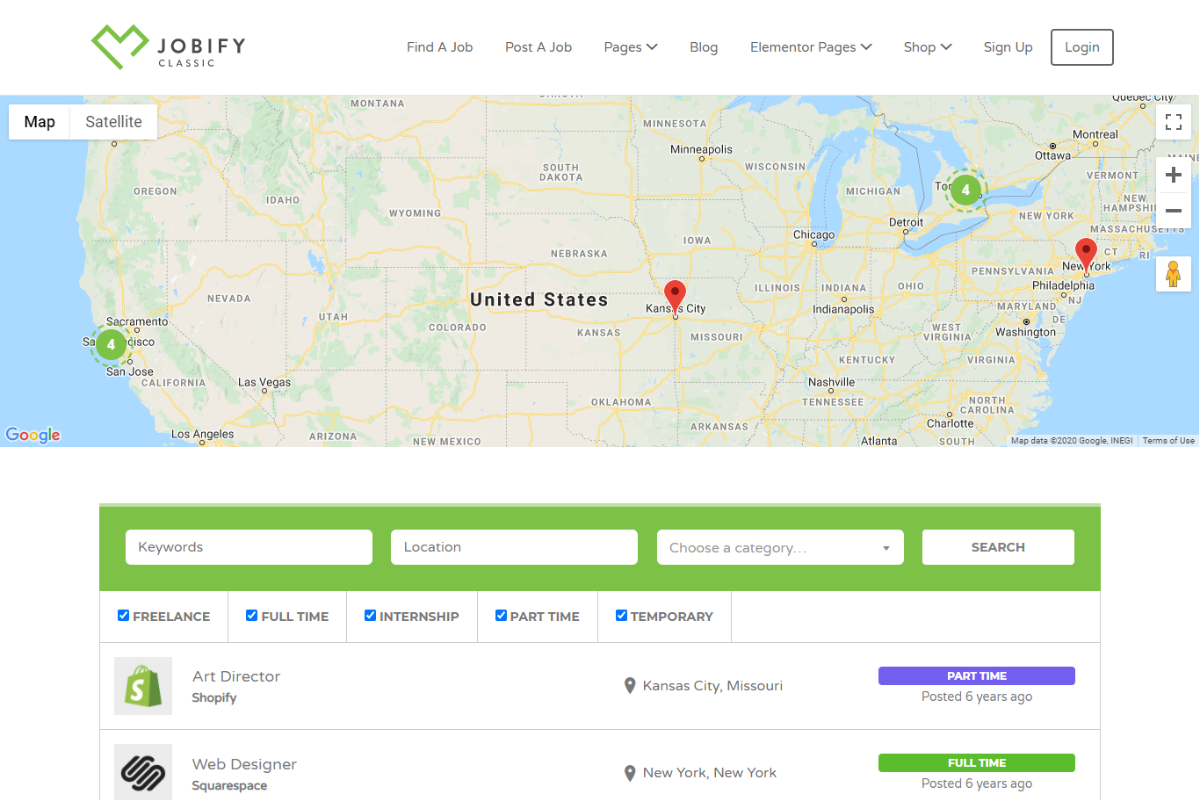This image is a detailed screenshot of the Jobify Classic website. It features a clean, white background. At the top left corner, there is a green heart-shaped logo followed by black text that reads "Jobify Classic." Next to it, there is a navigation menu with the following options: "Find a Job," "Post a Job," "Pages," "Blog," "Elementary Pages," "Shop," "Sign Up," and a "Login" button.

Below the navigation menu, there is an interactive color map of the United States with markers placed in Kansas City and New York. Directly underneath the map, there is a green banner containing dropdown menus and buttons labeled "Keyword," "Location," "Choose a Category," and a "Search" button.

The section beneath the green banner shifts back to a white background and contains tabs categorized by job type: "Freelance," "Full-Time," "Internship," "Part-Time," and "Temporary." Below these tabs, specific job listings are displayed. Among them are listings for an "Art Director" position at Shopify based in Kansas City, Missouri, classified as part-time and posted six years ago, and a "Web Designer" position at Squarespace located in New York, New York, listed as full-time and also posted six years ago.